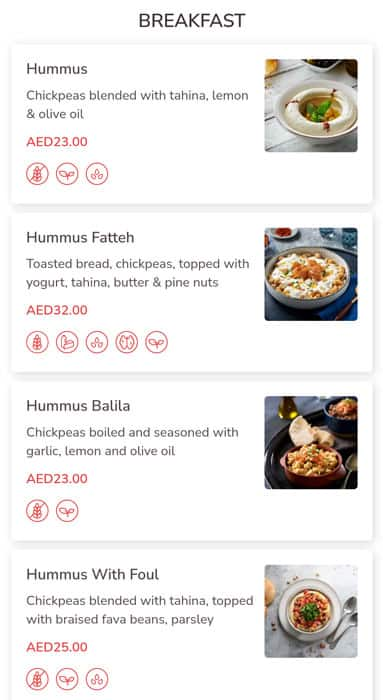This vertical rectangular image is titled "BREAKFAST" at the top in bold, black, all-capital letters. Below the title, the image is divided into four horizontal sections, each showcasing a different dish.

1. **Hummus**
   In the upper left corner, "HUMMUS" is written in bold black font. Underneath, in regular black font, the description reads: "Chickpeas blended with tahina, lemon, and olive oil." The price is listed below in red, all-capital letters: "AED 23.00." There are three icons beneath, each within a white circle outlined in red. The first icon features an item with a slash through it from the upper right to the lower left corner. To the right of the text is a vertical rectangular image of a bowl of hummus.

2. **Hummus Fatteh**
   Next, "HUMMUS FATTEH" is written in bold black font, followed by the description in regular black font: "Toasted bread, chickpeas topped with yogurt, tahina, butter, and pine nuts." The price is listed in red, all-capital letters: "AED 32.00." Five red-circled icons are positioned beneath the price. To the right of the text is an image of a bowl of hummus fatteh.

3. **Hummus Balila**
   The third section features "HUMMUS BALILA" in bold black font. The description below, in regular black font, reads: "Chickpeas boiled and seasoned with garlic, lemon, and olive oil." The price is displayed in red, all-capital letters: "AED 23.00." Two red-circled icons are positioned below the price, with the first icon featuring a line through it. Adjacent to the text is an image showing a bowl of hummus balila with pita bread placed above it in the picture.

4. **Hummus with Fowl**
   The last section is titled "HUMMUS WITH FOWL" in bold black font. The accompanying description in regular black font states: "Chickpeas blended with tahina, topped with braised fava beans, parsley." The price, in red, all-capital letters, is "AED 25.00." Below it are three red-circled icons, with the first one featuring a line through it. To the right of the text is an image showcasing a bowl of hummus with fowl and two spoons to the right of the bowl.

Each dish is visually represented next to its description, offering a detailed and appetizing preview of the breakfast options.